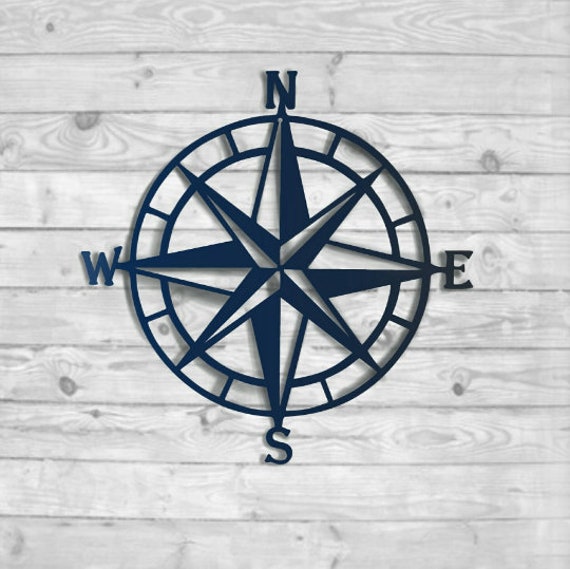The image features a detailed decorative compass ornament, seemingly made of cast iron, displayed against a pale grey, white-washed wooden plank wall with horizontal boards and visible wooden knots. The ornament is circular, designed in navy blue, and prominently displays the letters N, E, S, and W indicating the cardinal directions at the outer edge. The central design includes an eight-point star formed by a four-point star with a smaller, perpendicular four-point star overlaid. The points of the stars are partially filled with a black material, creating a striking contrast. Surrounding the star, the compass has two outer rings, giving the appearance of a steering wheel.